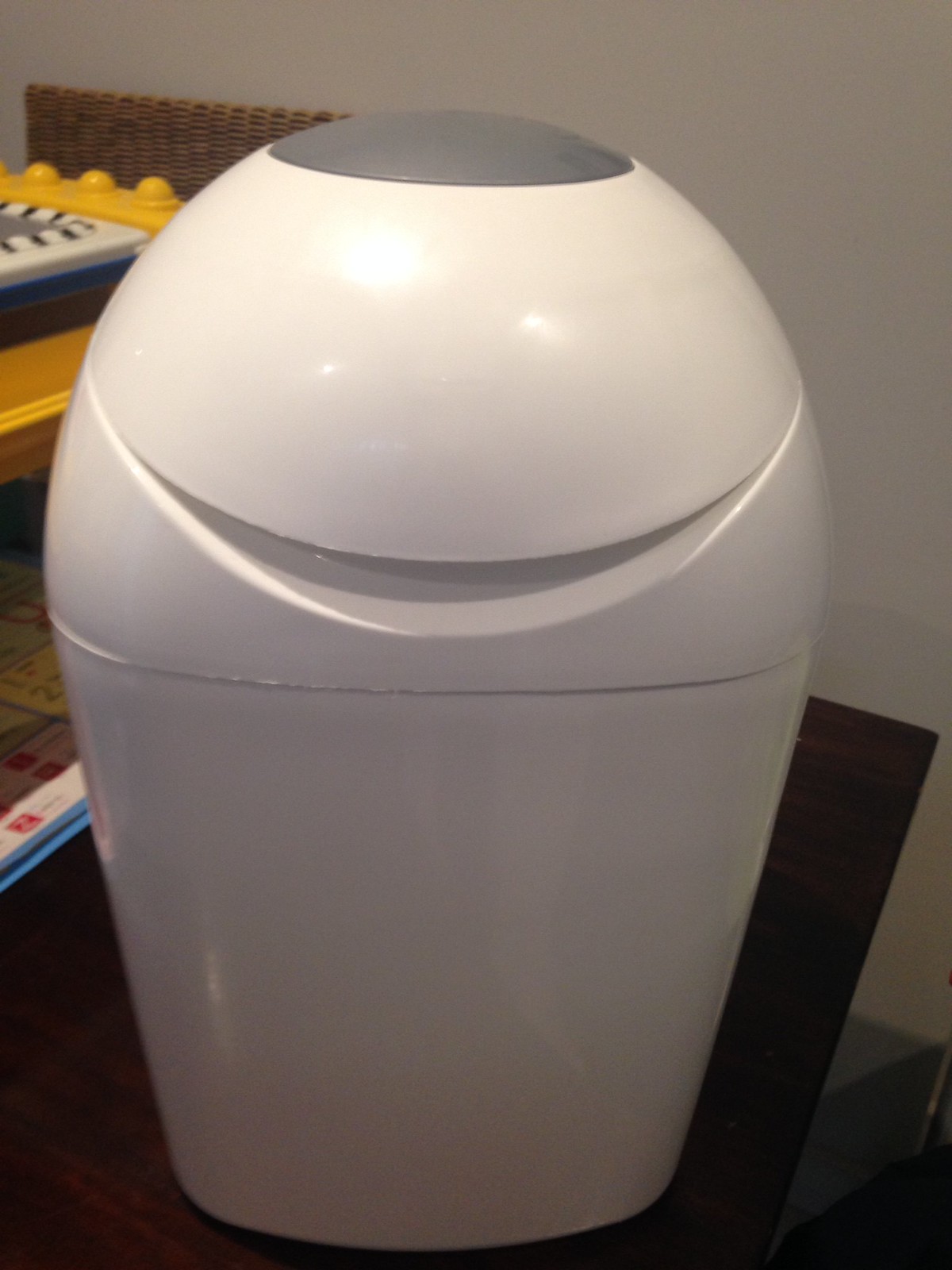The image features a bright white, miniature plastic trash can with a sleek, inverted trapezoid design. The can sits prominently on a dark brown wooden desk. It's fitted with a grey circle on its dome-shaped lid, which swings open to allow waste disposal. Behind the trash can, a variety of items rest on a shelf, including educational materials and toys, notably yellow plastic pieces resembling Lego blocks. A blue and white plastic item, a board game which could be Monopoly, and a wicker object are also visible. The wall in the background is white, contrasting with the intricate scene in front.